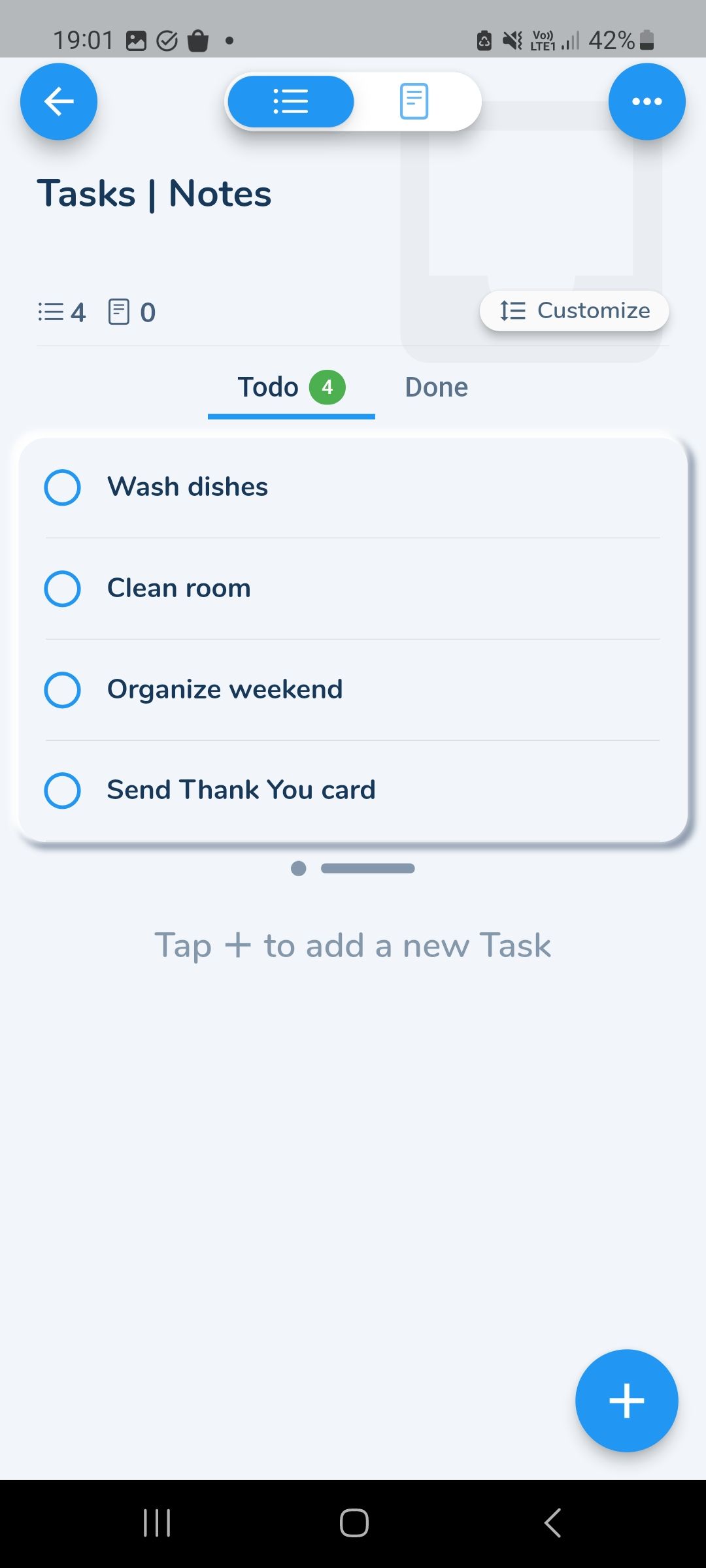The background of the image features a gradient transitioning from a pretty light blue at the top to black at the bottom. On the lower-left corner, there are three horizontal white lines. Nearby, there is a black square framed by a white border, and an arrow points to the left. Just above the tip of this arrow, a blue circle with a white plus sign is visible. 

Moving upwards, in light gray text, it indicates, "tab plus to add a new tab." Continuing further up, there is a gray circle with a gray oval, followed by a larger light blue square with four circles outlined in blue. Next to each of these circles, there is black text with clickable options: "Watch this" next to the first, "Clean room" next to the second, "Organize weekend" next to the third, and "Send thank you card" next to the last.

Above this, there is black underlined text stating "To Do," accompanied by a green circle containing a white number four. Adjacent to this, in gray text, is the word "Done." A thin line runs horizontally across the image above these elements.

On the left side of this line, there are three horizontal lines and a small circle, followed by the number four. Next to this, an icon resembling a piece of paper is displayed alongside the number zero and the word "Customize." In the top-right corner of the image, the current time shows as 19:01 and the battery is at 42% charged.